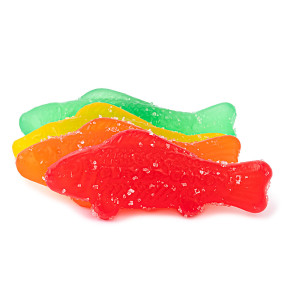The image depicts a vibrant, multi-colored circular arrangement of gummy fish candies with no specific border, set against a plain white background. The candies, resembling Swedish Fish, are coated in a fine layer of sugar, giving them a dusted appearance. The assortment features a variety of colors including blue, green, yellow, orange, and red. Each gummy fish remains intact, contributing to the overall texture without appearing bent or broken. The fish are tightly packed together, forming a spherical ball. This cluster draws attention to the different colors intermingled, creating a visually striking confectionery sculpture with sugar crystals glistening across their surfaces.